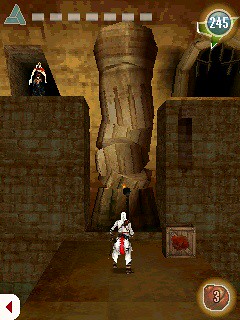This is a pixelated screenshot of a mobile game, possibly from the Assassin's Creed series, featuring a white-hooded character in white robes with a distinctive red line running down the back. The scene is predominantly in dark brown and gray hues, depicting two large, castle-like stone walls on the left and right sides, with a crumbling tan column between them. The upper left of the image shows a triangular shape with gray hashed lines. In the bottom left corner, there is a red back arrow, while the bottom right corner displays a bomb-like icon with the number three on it. A blue circle in the upper right corner shows the number 245 in white letters. A large wooden box with a red mark is positioned in front of the right pillar. The setting includes a big concrete platform, and in the middle, the white-robed character seems to be looking at a black wrought-iron candle holder with a flame. Above the scene, there's another figure with elements of red, white, and blue, positioned on a stone ledge, partially obscured by gray dashes and a green triangle at the top of the image.